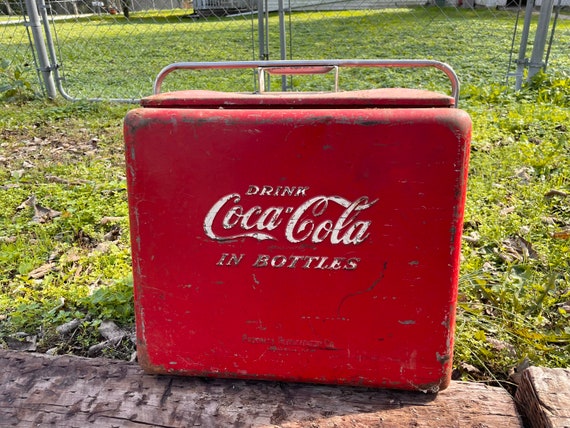The photograph captures an outdoor scene featuring an old, battered red Coca-Cola cooler, prominently displaying the iconic "Drink Coca-Cola in Bottles" logo, which is partially worn off. The cooler, likely from the 1950s or 60s, exhibits signs of heavy wear with rust and scratches revealing the metal beneath the faded paint. It's equipped with a silver metal handle that arches over the top and a red cap. The cooler is positioned slightly ajar, perched on a flat surface that appears to be either wood or stone, set amid a well-maintained grassy area. In the background, a chain-link gate fence is visible, indicating it's a closed gate. Beyond this, hints of a building can be seen at the very top of the image, under a bright and clear sunny sky, completing the nostalgic, rustic atmosphere of the scene.